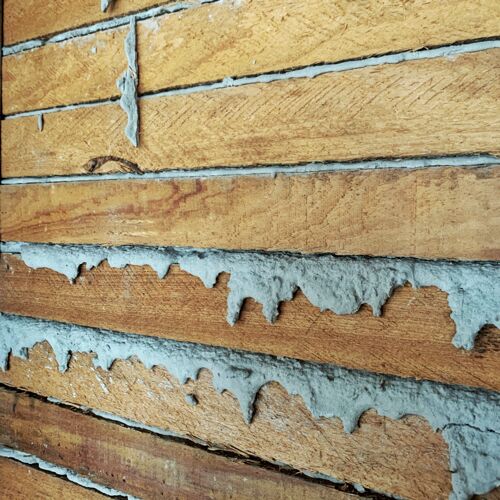This close-up photograph captures a section of an exterior wall composed of horizontally laid, rough, light-colored wooden boards. The wood displays signs of aging, with visible striations and weathering, creating a textured and natural appearance. Nestled between the gaps of these six slat boards are streaks of frost or snow, possibly mixed with other residues such as mold or dust, that have seeped through from the outside. Some of this residue has hardened and dripped along the surface, creating patterns that accentuate the rustic aesthetic of the wall. One of the boards notably features half of a knot hole, adding to the rugged charm. The close-up nature of the shot prevents identification of the larger structure, focusing instead on the intricate details and interplay of natural elements on the wood.